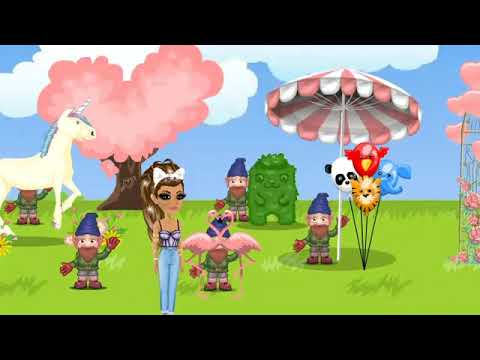The image appears to be a vibrant, whimsical scene potentially from digital art or a video game, bordered by black horizontal lines on the top and bottom. It features a cartoon-like world with bright green grass beneath a vivid blue sky dotted with fluffy white clouds. Dominating the foreground is a slender young woman with long brown hair adorned with white sparkles, wearing blue jeans, a white corset-style tank top, and a white cat ear headband. She has light skin and large eyes.

Scattered throughout the scene are several gnome figures dressed in green jackets, red gloves, blue hats, brown beards, and brown shoes. One gnome is playfully hiding behind two pink flamingos near the woman, while another stands under a pink and white striped umbrella, surrounded by animal-shaped balloons resembling a panda, an elephant, a cheetah, and a bird.

In the background, a heart-shaped tree with a brown trunk and vibrant pink leaves adds a romantic touch to the fantastical setting. Nearby, a majestic white unicorn with blue and purple hair and a twisted horn on its head grazes. Additional details include what appears to be a terraced archway adorned with pink flowers to the right and a fuzzy, grass-like character in the center, gazing directly at the woman. The overall scene exudes a sense of playful fantasy with a diverse array of quirky elements.